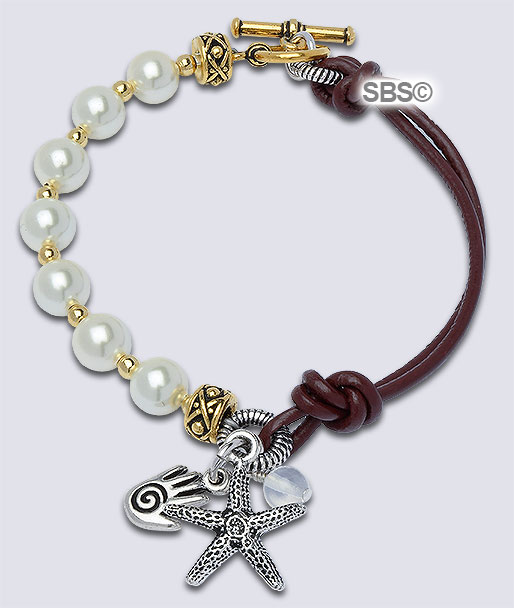This is a detailed color photograph of a handmade bracelet highlighting various materials and charms. The bracelet features a dual design: the left side comprises round white pearls interspersed with gold-colored beads, including two thicker gold-and-black ring-like beads. On the right side, the bracelet is fashioned from brown leather string with a gold clasp. Central to the bracelet are silver charms—a starfish and a hand with a black swirl in its center—along with a small transparent bead. Positioned at the bottom of the image are the starfish and hand charms, with the pearls on the left and the leather string on the right. The text "SBS copyright" is visible in the top right corner. The overall color palette includes pearl white, gold, metallic gray, and dark burgundy, suggesting an advertisement style presentation for this intricate wristband.